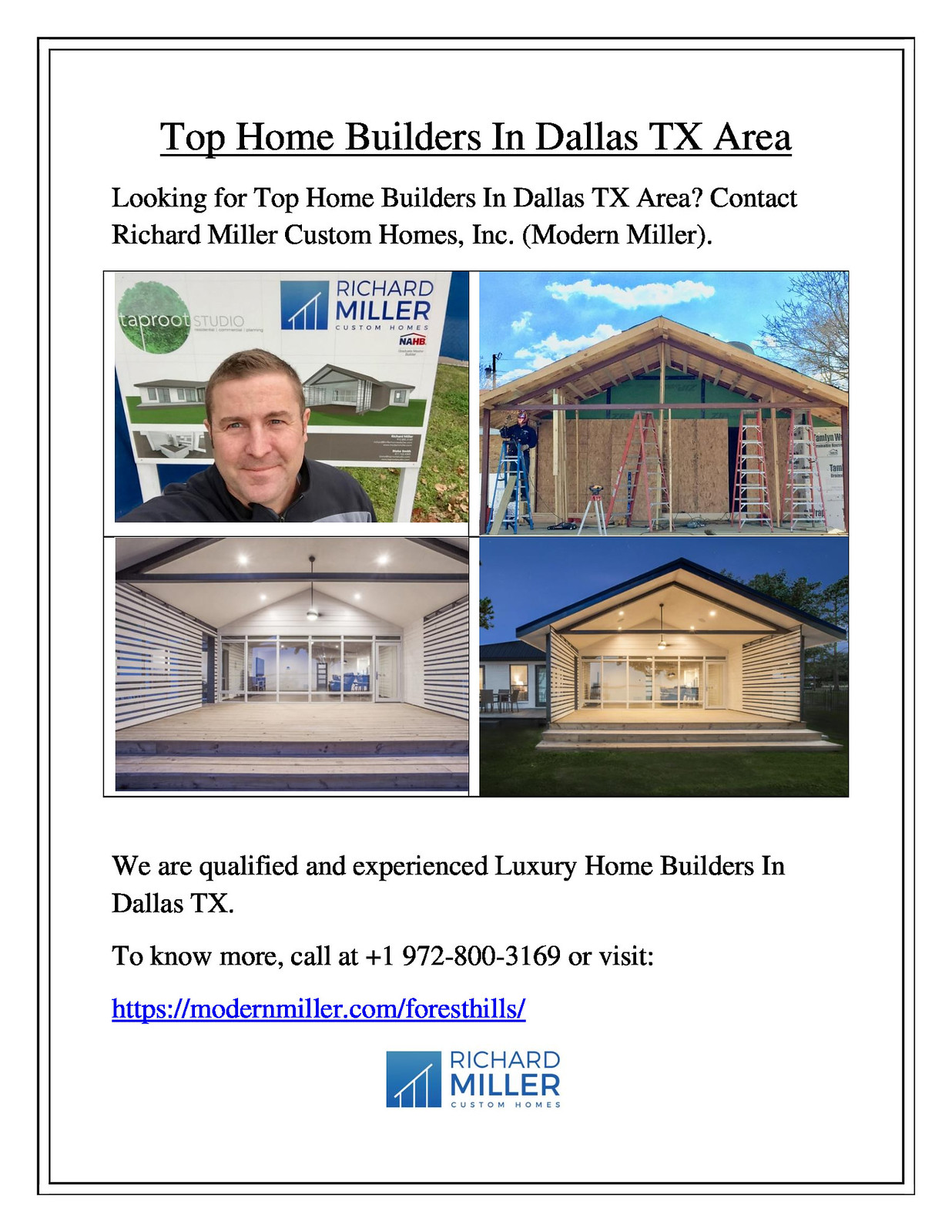This detailed rectangular advertisement for Richard Miller Custom Homes Inc., also known as Modern Miller, is designed to attract potential clients in the Dallas, Texas area. The ad features a double black border on a white background, with the central content comprised of four key photographs and informative text. 

The header, prominently displayed in large, underlined text, reads "Top Homebuilders in Dallas, Texas Area." Below it, in slightly smaller text, it asks, "Looking for top homebuilders in Dallas, Texas area?" followed by the contact information: "Contact Richard Miller Custom Homes Inc. (Modern Miller)." 

The four photographs are centered within the ad, showcasing the work and persona of Richard Miller. The top left photo features Richard Miller himself, a friendly-looking, middle-aged Caucasian man with light brown hair, standing in front of a sign that reads "Richard Miller." Next to this, the top right photo displays a partially built home, highlighting the wooden framework, ladders, and workers actively engaged in construction. 

The bottom left image presents the interior of a completed home, characterized by a spacious room with blue and white horizontally striped walls, a white ceiling, and a white floor, devoid of furnishings. The final photo, at the bottom right, captures the exterior of a finished home, providing a view from the yard of the meticulously constructed building.

Ensuring potential clients of their qualifications and experience in luxury home building, the ad states, "We are qualified and experienced luxury homebuilders in Dallas, Texas." For more details, it provides a contact number: 1-972-800-3169, and a website link: https://modernmiller.com/FORESTHILLS/.

At the bottom of the flyer, a simplified blue and white logo alongside the text "Richard Miller Custom Homes" reinforces the brand identity. The color scheme of the ad includes black, white, gray, peach, yellow, tan, brown, blue, and green, adding a visually appealing touch to the informative layout.